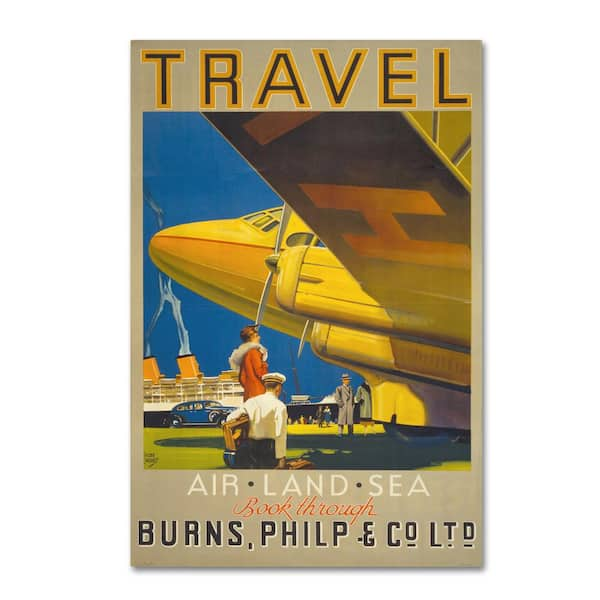This vintage-style poster serves as an advertisement for a travel agency, titled "Travel." At the top of the beige background, the word "Travel" is prominently displayed in a black font with a gold outline. Below it, a sequence of texts appear: "Air, Land, Sea" in white, followed by "Book Through" in orange cursive, and finally, "Burns, Philp, and Co., Ltd" in bold black.

The central focus of the illustration is a detailed, 1950s-era yellow airplane, viewed from underneath. This aircraft features two propellers positioned where the wings meet the fuselage, with the plane angled towards the left. Prominently displayed on the plane's wing is an orange letter 'H'. 

Below the airplane, three people are depicted: a pilot in traditional gear with a white shirt and captain's hat, carrying luggage; a woman in an orange fur coat; and a man in a grey trench coat. Additionally, another pilot in a red bomber jacket with a fur collar can be spotted. In the background, to the left, a blue car, possibly a Rolls Royce or similar model, is parked. Further back, a large, Titanic-like steamship with two smoking orange chimneys stretches across the scene, emphasizing the various modes of transportation.

The entire scene is set under a clear blue sky, with a few individuals seen in the distant background, contributing to the overall nostalgic and classic travel theme of the poster.